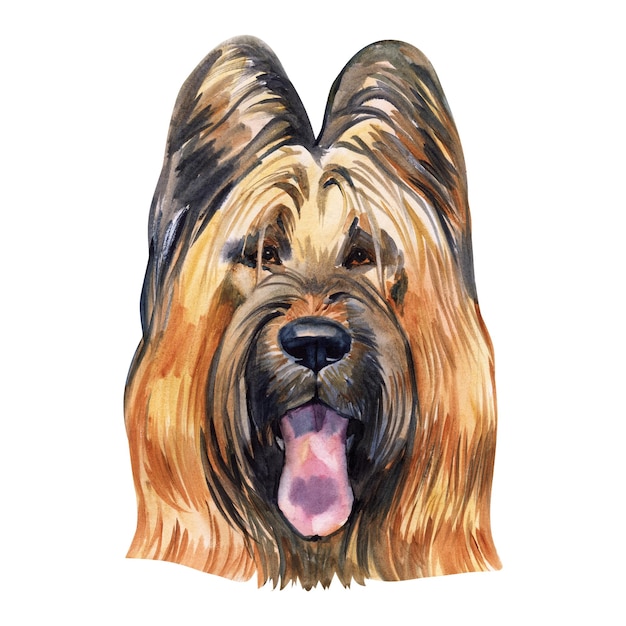The image depicts a meticulously painted close-up of a dog's face, set against an entirely white background. The dog, bearing a striking resemblance to a sheepdog with its characteristic long hair, stares directly at us with expressive brown eyes that possess black centers. Its face showcases a gradient of brown shades, starting with light brown fur above the eyes, transitioning to a darker brown around the snout and cheeks, and then back to light brown towards the bottom. The large, prominent ears stand erect, displaying a mix of black, gray, and brown hues. The dog's nose is black, and just underneath it, patches of darker fur are visible. Its mouth is open, revealing a pink tongue speckled with purple, adding a playful touch to its appearance. The fur framing the face is long and slightly wavy, cascading down either side without a defined border, emphasizing the softness of the dog's coat. This detailed artistic rendition captures the dog's endearing features and its engaging, lively presence.